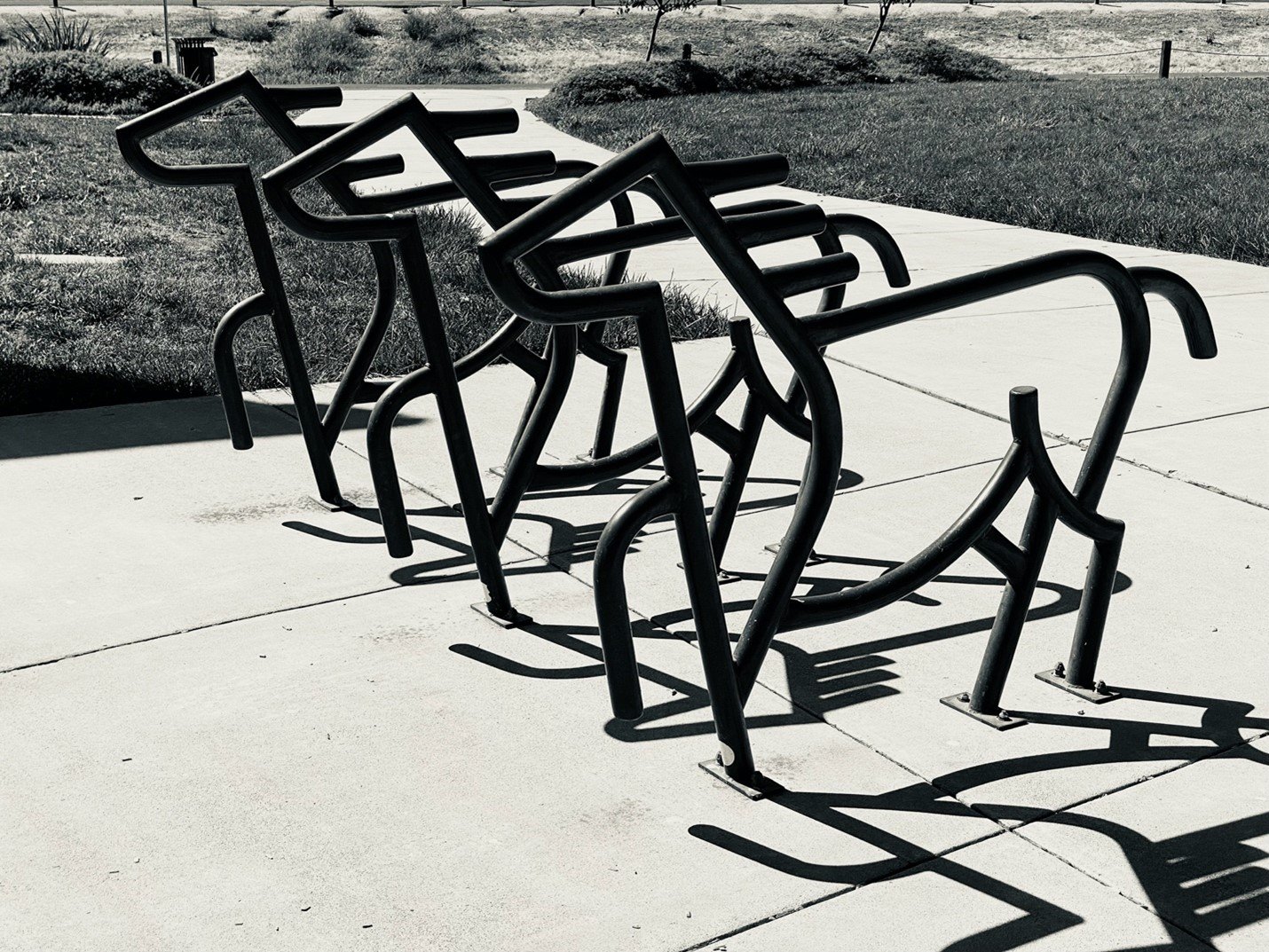The black and white photograph depicts a piece of functional yet abstract outdoor art. It features three metal outlines of horses, each bolted onto separate U-shaped legs that anchor them to a flat concrete pedestrian pathway. These horse frames, with their bars bent to mimic manes, are arranged parallel to each other, all facing towards the left side of the image. The horses create intricate shadows on the sidewalk, indicating a bright day. The background features a short-cut grassy area flanking both sides of the pathway, with the grass mound blending into extensive flatlands culminating in a left-to-right road in the distance. The overall scene exudes a sense of open space and artistic integration into the environment, hinting at the pieces' potential function as hitching posts for horses or bicycles in this locale.